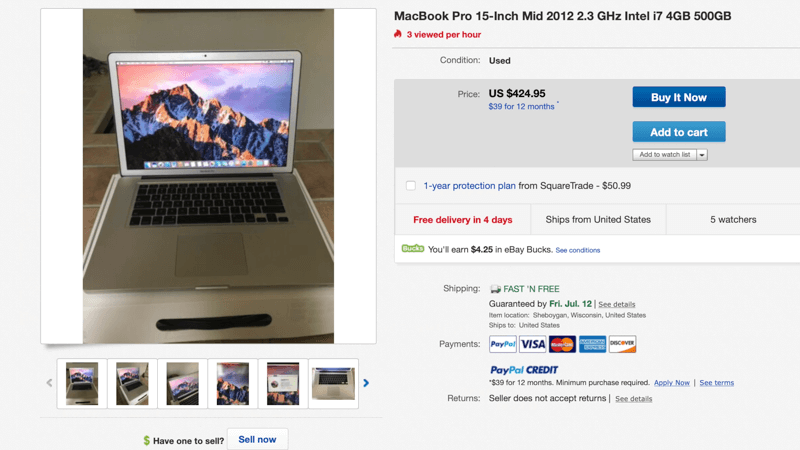A detailed descriptive caption for the image:

"This is a screenshot of an eBay listing page for a MacBook Pro. The item up for auction is a mid-2012, 15-inch MacBook Pro featuring a 2.3 GHz Intel i7 processor, 4 GB of RAM, and a 500 GB hard drive. The condition of the laptop is listed as 'Used.' Notably, the listing highlights in red text with a small fire icon that 'Three viewed per hour.' The price is set at $424.95 USD, with an option to pay $39 monthly for 12 months, as indicated in blue text. There are two prominent buttons to the right: a blue 'Buy It Now' button and a lighter blue 'Add to Cart' button, with an 'Add to Watchlist' dropdown menu below them.

The left side of the page displays a photo of the open MacBook Pro, showcasing its silver body, black keyboard, and screen with a mountain background. Thumbnails below this main image provide additional views of the laptop. Below these thumbnails is a prompt that reads 'Have One to Sell? Sell Now.'

Additional details on the page include a 'Fast and Free Shipping' notice, guaranteeing delivery by Friday, July 12. The item is currently located in Sheboygan, Wisconsin, and is available for shipping within the United States. Accepted payment methods include PayPal, Visa, MasterCard, Amex, Discover, and PayPal Credit."